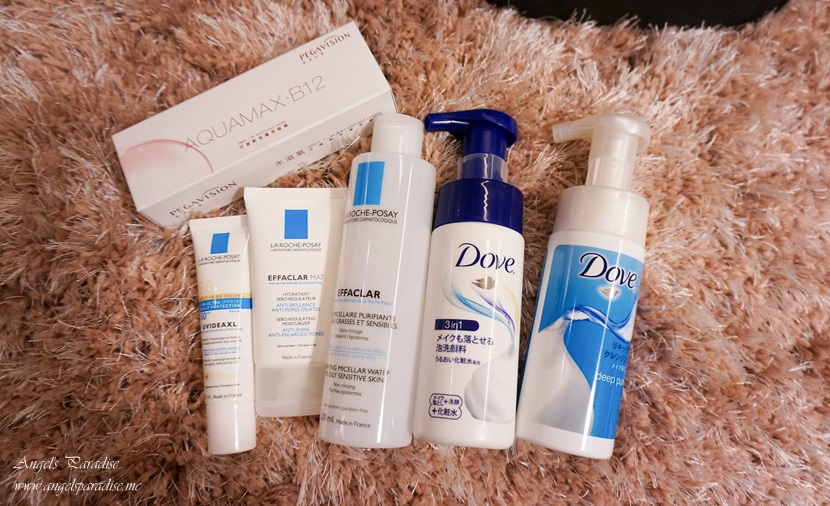The image depicts a collection of beauty products meticulously arranged on a mauve pink, shaggy bathroom rug. In the bottom left corner of the rug, an insignia that reads "Angels Paradise" is elegantly inscribed in a fancy, curvy font, accompanied by the website "www.angelsparadise.me". The beauty products, which include a variety of bottles and a box, are prominently displayed across the rug.

On the left side of the arrangement, there are two Dove products in pump-style bottles. The leftmost bottle is predominantly white with blue accents and displays the Dove logo alongside a "Three in One" label. The adjacent Dove bottle, also blue and white, features Asian characters, indicating a possible Asian origin.

Further to the left, three additional products are visible. These include a larger bottle and two smaller squeeze bottles, which bear the label "Effaclar", suggesting they are likely skincare products. Above them sits a white, rectangular box labeled "Aquamax-B12" with the brand name “Pegavision” in the right corner. This box contains Asian characters and has a pink tint that complements the mauve rug below.

This detailed arrangement of beauty products showcases a thoughtful alignment, emphasizing the aesthetic appeal of both the items and the backdrop.